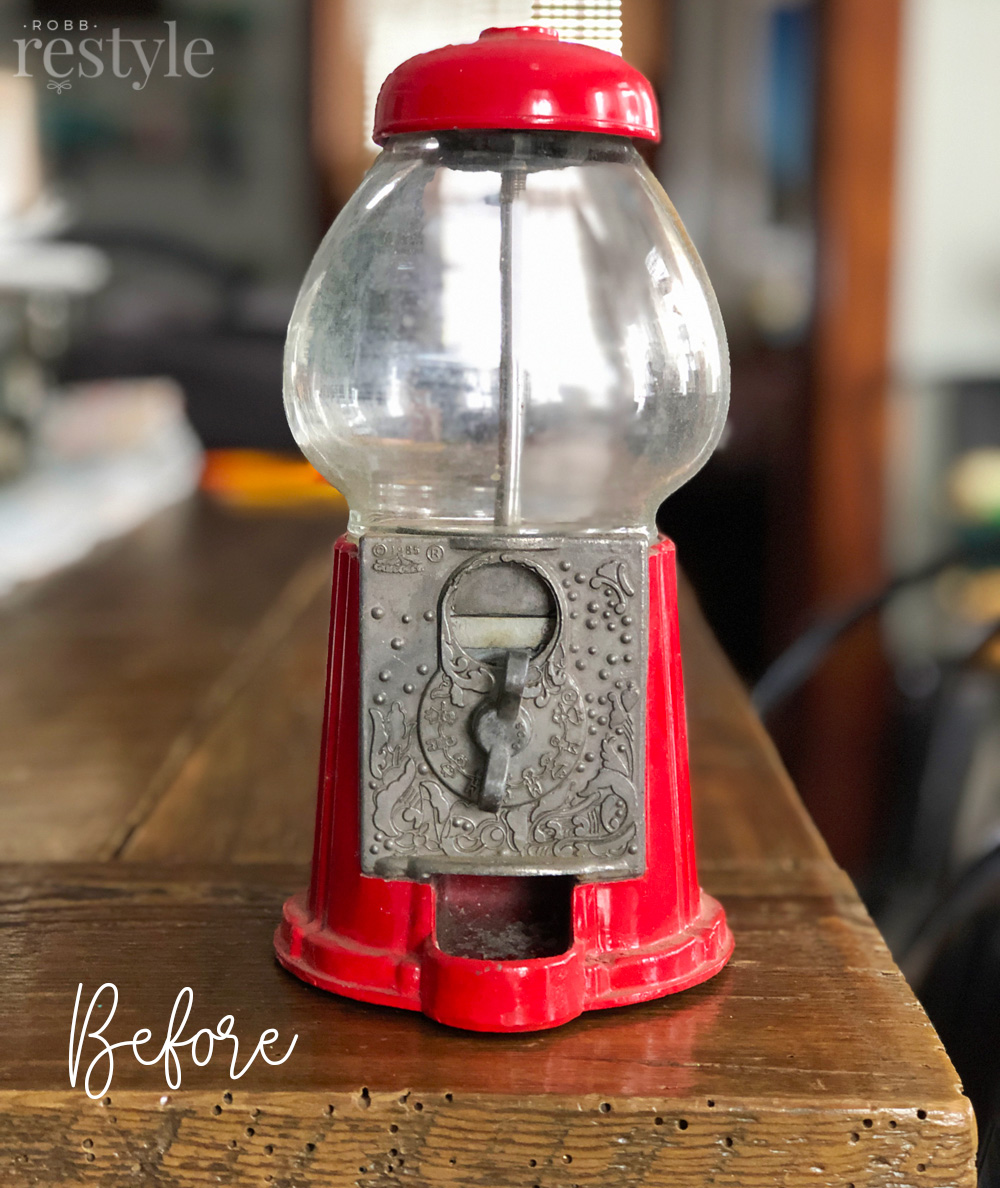This image is a detailed photograph of an old, empty gumball machine poised on a worn, vintage wooden table. The gumball dispenser features a red, dome-shaped cap and a matching red base, with a clear, cylindrical midsection. The metal handle at the front—a dull gray wingnut—is designed for turning to dispense candy. The glass is slightly dusty and cloudy, implying age and wear. Notably, corrosion is visible on the metal parts, and grunge marks the glass. Behind the gumball machine, elements of an indoor setting are barely discernible, including a wooden paneled section on the right, a white wall, and a daylight-illuminated window that reveals something blue and gray on the left. For added context, the top of the image reads "Rob ReStyle" in gray letters, while the bottom features the word "Before" in white script, suggesting the machine is due for restoration.